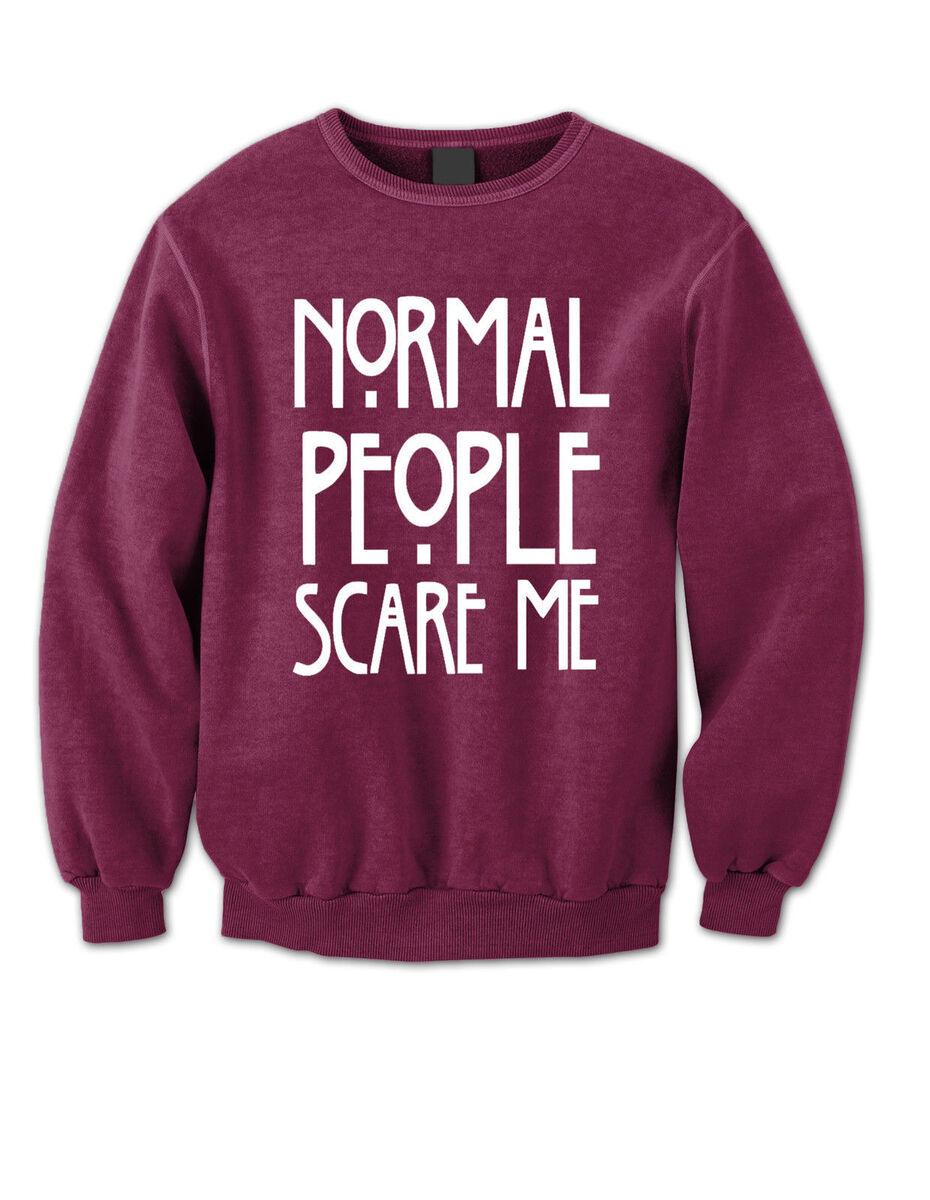This image is a full-color, square photograph of a burgundy (dark red) long-sleeved sweatshirt displayed against a plain white background. The sweatshirt is slightly rumpled, with visible air pockets, and features banded cuffs and a bottom hem. A black tag is noticeable at the back of the standard neckline. Across the chest of the sweatshirt, in large, capitalized white letters reminiscent of the American Horror Story font, is the phrase "Normal People Scare Me." Notably, the "O" in "Normal" and "People" includes a dot underneath, the "A"s in both "Normal" and "Scare" have two crossing lines, and the "E"s have irregular shapes.